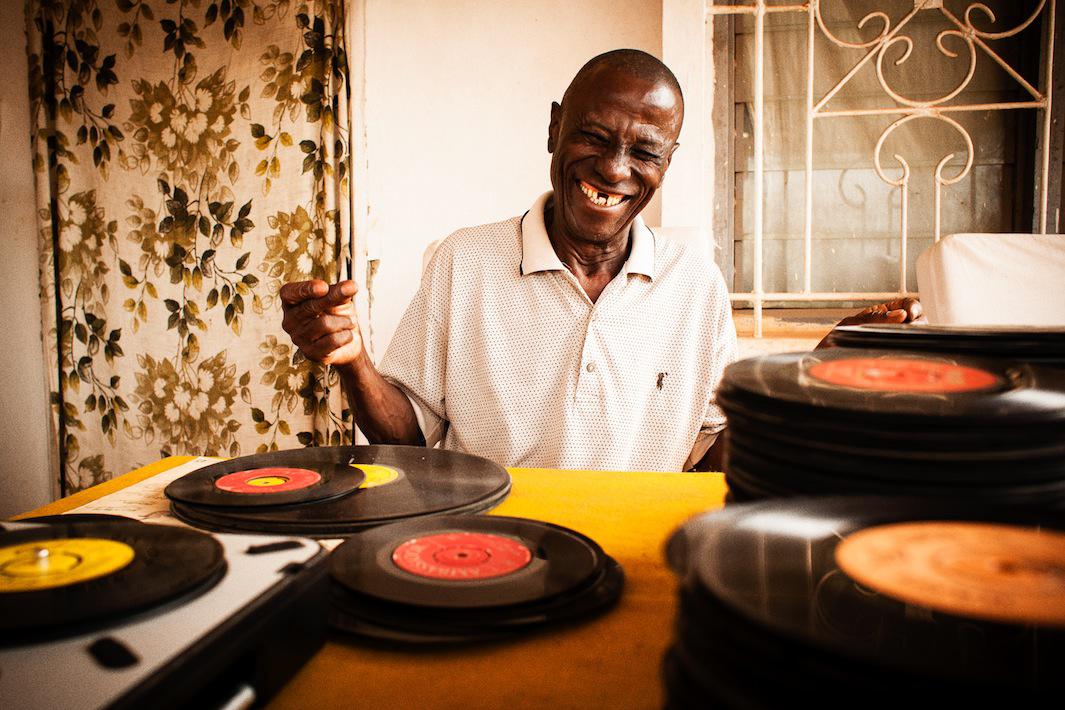This is a captivating image of an older black man with dark brown skin, bald head, and a noticeable gap in his front teeth, laughing joyfully with his eyes closed. He is dressed in a beige-colored polo shirt adorned with a Ralph Lauren emblem and has his right hand raised, as if he is snapping his fingers and dancing to the music. He sits before an orange-hued table, stacked high with numerous records, the majority of which have red labels, although some feature yellow labels. Positioned to his left is a black and silver record player with a black record spinning, marked by a yellow sticker in the center.

The background behind him reveals a beige wall and to his right is a vertically hanging beige curtain with green leaf patterns. To his left, a window is visible with white wrought iron embellishments, resembling a security fence, and partially covered by a fabric with floral patterns in browns and greens. The setting evokes a warm, nostalgic atmosphere, enriched by the details of the room's decor and the man's infectious, carefree enjoyment.